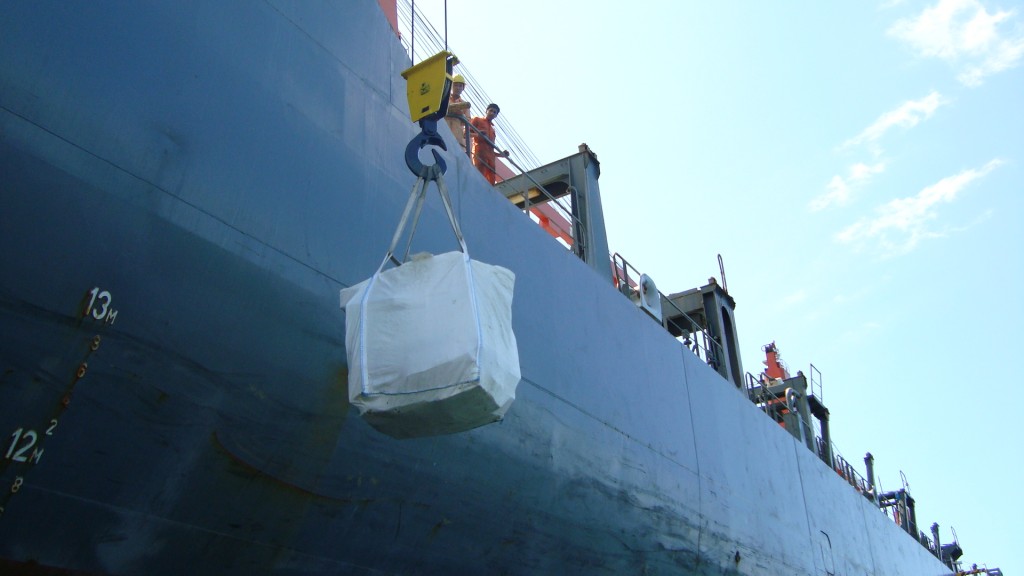The image is a detailed outdoor photograph capturing part of the port side of a large, tall ship in daylight. The sky to the right of the image is partly cloudy. Dominating the scene is the ship's hull, marked with the numbers "12" and "13M" near the bottom left, and the vertically arranged letters "2MH." A yellow metal piece with a hook extends from the ship's side, lifting or lowering a white-wrapped box whose contents are unknown. On the deck above, secured behind safety netting, stand two people: one on the left wearing a yellow safety helmet, and the other on the right in reddish-orange clothing, focused on the cargo. The photograph does not encompass the entire ship but showcases an expansive view of its side and part of its deck, without any additional people clearly visible toward the distant end.